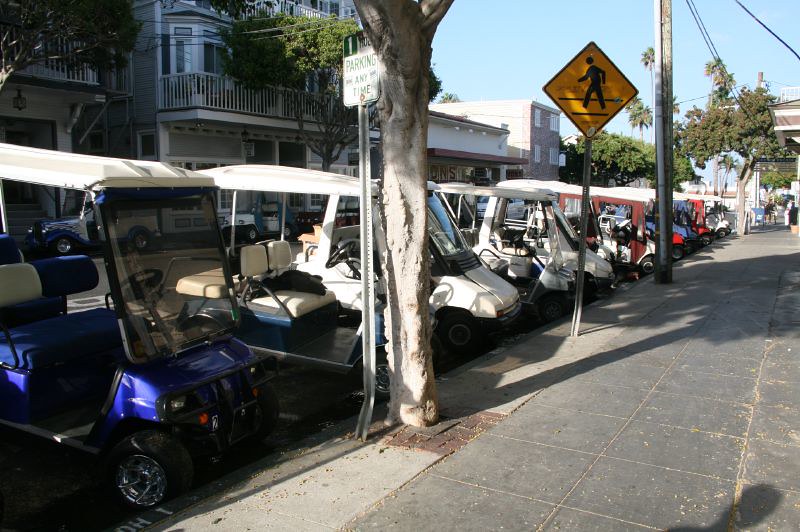This image captures a vibrant street scene during daylight, showcasing a well-maintained urban avenue beneath a clear blue sky adorned with palm trees. The street is paved with gray bricks, adding texture to the scene. Along the sidewalk, there is a distinct row of variously colored golf cart-like vehicles, though larger in size. The closest one is blue with a white top and blue-and-white seats, while others stretch further down the street. Each vehicle is parked tightly against the curb, fronts facing inward, creating a neat lineup.

Parallel to this sidewalk runs an assortment of buildings, including apartments with white-banistered balconies and a distinctive tall gray house-like structure with a balcony porch. Power lines and cables crisscross above, contributing to the urban feel. This bustling scene is punctuated by several signs: a prominent yellow pedestrian crossing sign, a "no parking" sign near a tree, and another sign indicating parking regulations. The trees, bordered by brick bases, provide a natural touch, complementing the modern cityscape.